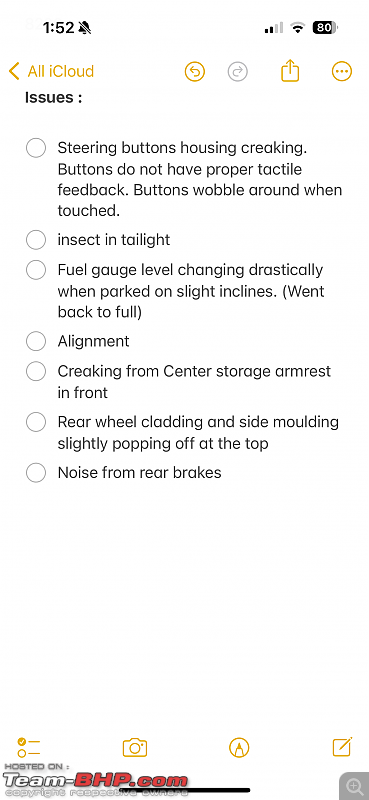**Caption:**

The image displayed on a smartphone has a vertical orientation with a white computer screen as the background. In the top-left corner, the time reads 1:52, accompanied by a bell icon with a slash through it, indicating that notifications are muted. The top-right corner shows a signal with two bars, a weak Wi-Fi connection, and an 80% battery life.

Below the status bar, on the left, there's a yellow arrow pointing left labeled "All iCloud" next to a gray arrow pointing right. These are beside the share button and a circle containing three horizontal dots.

Directly underneath "All iCloud" in bold black text, the heading "Issues:" is followed by a list of seven unfilled circles with accompanying descriptions:
1. **Steering Button**: Buttons housing creaking. Buttons do not have proper tactile feedback. Buttons wobble around when touched.
2. **Insect and Tail Light**
3. **Fuel Gauge**: Fuel gauge level changes drastically when parked on slight inclines. It sometimes returns to full.
4. **Alignment**
5. **Creaking from Center Storage**: Armrest in front.
6. **Rear Wheel Cladding and Side Molding**: Slightly popping off at the top.
7. **Noise from Rear Brakes**

At the bottom of the list, the text "TeamBPH.com" is followed by a camera icon, an area for additional writing, a magnifying glass, and a pencil icon.